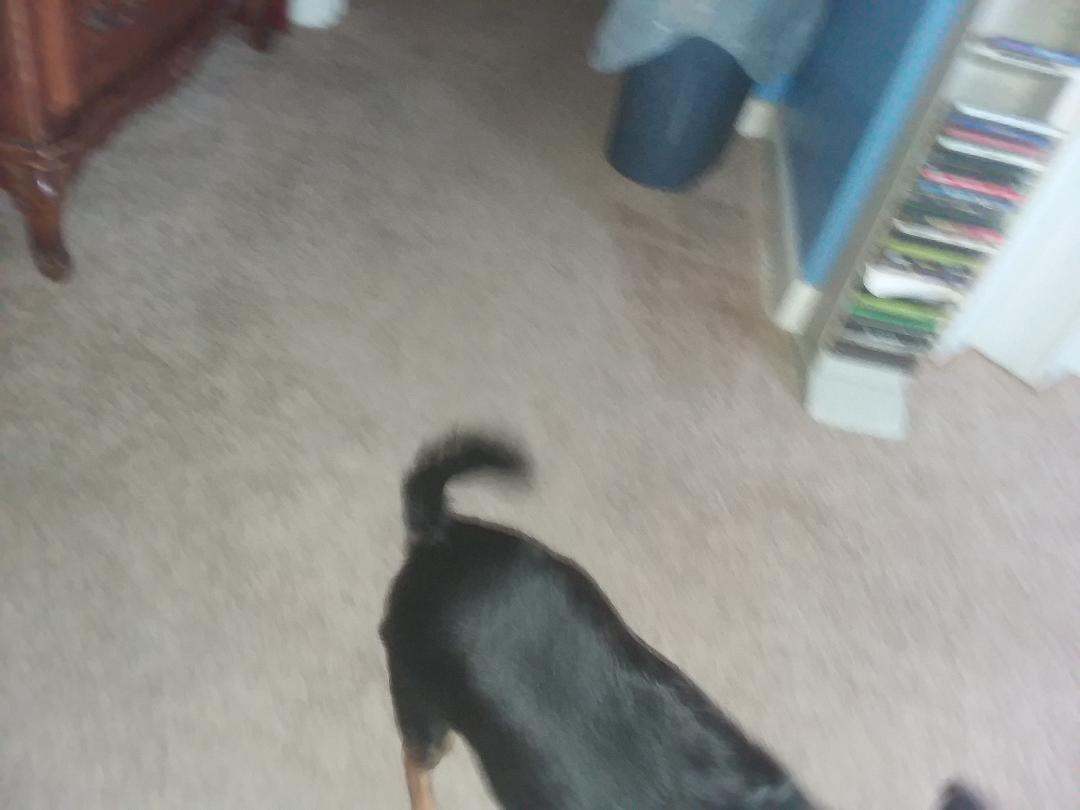A blurred color photograph captures a bird's-eye view of a room with beige carpeting. In the lower right and center of the image, a black dog is partially visible, shown from its front shoulders to its tail. The dog appears to be happy, indicated by its tail arched over its back to the right. The tip of one ear is also visible in the lower right corner. Towards the upper right corner of the photograph, a white shelf, slightly tilted, holds DVD or CD cases against a blue wall. A blue plastic trash can with a white trash bag folded over the top is located in the upper left corner. Additionally, the bottom half of the lowest drawer of a brown wooden dresser can be seen in the upper left area of the image.